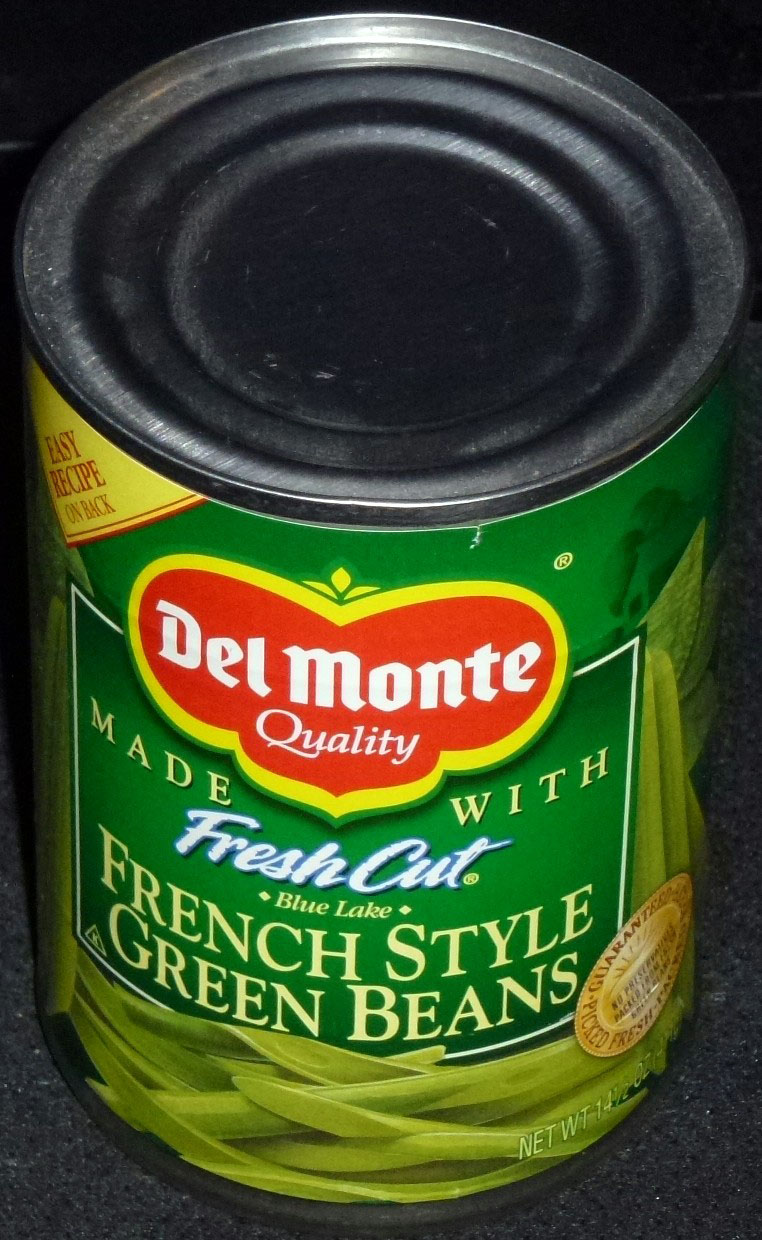The image is a detailed photograph of a standard round aluminum can of Del Monte green beans, positioned vertically on a dark gray countertop in a kitchen. The can features a green paper label with a realistic photograph of green beans at the bottom. Prominently displayed at the top of the label is the red and white Del Monte quality logo with a yellow surround on a green background. Below the logo, the label reads "Made with fresh cut Blue Lake French style green beans" in light green color. Additionally, there’s a small gold triangle in the top corner of the label, indicating an "easy recipe on the back." The can, which requires a proper can opener to open, is slightly dirty on the top but otherwise appears as a typical grocery store item. There is no other object visible in the image.